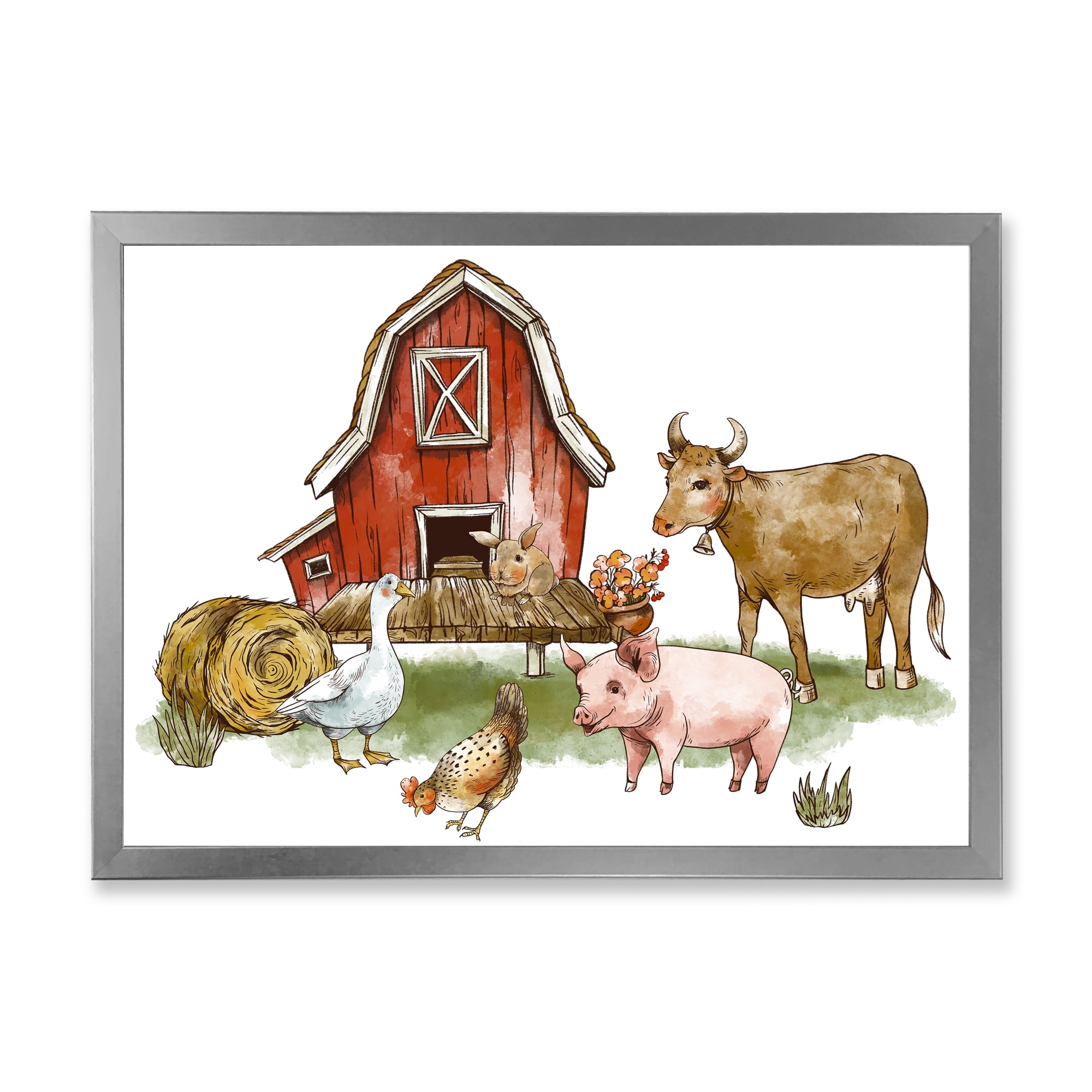This is a detailed illustration of a farm scene, presented as a framed print against a white background. The thin frame surrounding the image is gray. At the center of the scene stands a small red barn with white paneling and barn doors, elevated on stilts. On its porch sits a brown rabbit, alongside a little wooden table. Nearby, there is a bowl filled with flowers and a smiling pink pig standing on a tuft of grass. In front of the pig is a chicken, with a red comb and brown feathers, pecking the ground. To the right, a white goose with webbed feet and a pointed bill looks on, with a roll of hay beside it. A brown cow with horns and a bell around its neck adds to the pastoral charm. The entire illustration, rendered in watercolor, captures the whimsical essence reminiscent of a children's book illustration, making it an ideal piece for a child's room.